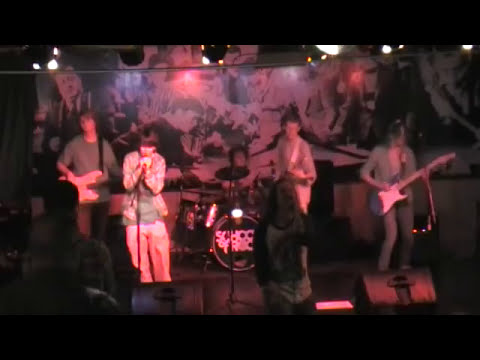This image, captured from a distance, depicts a live concert on a dimly-lit stage, possibly inside a small club or venue. The overall poor quality of the image suggests it might be a photo of someone's TV screen or a printout. The backdrop of the stage features a black and white collage of various musicians, enhanced by stage string lighting and overhead lights. A warm pinkish-red glow illuminates the band members.

There are six performers on stage: two singers, two guitarists, a bass player, and a drummer. The drummer's black drum set prominently displays the white text "School of Rock" on the bass drum. From left to right, the band members include a bass player in a light green shirt and dark pants, a singer in a light flannel jacket, another guitarist partially obscured by someone in the audience, and another guitarist or possibly a third performer in a light green shirt and jeans playing a white and blue guitar. 

In the audience, three individuals are visible: one person turned toward the camera wearing a white shirt over a black long-sleeve shirt, a balding gentleman with glasses, and another individual with dark hair in a flannel shirt. The cozy atmosphere, combined with the intimate setting, suggests a small venue concert experience.